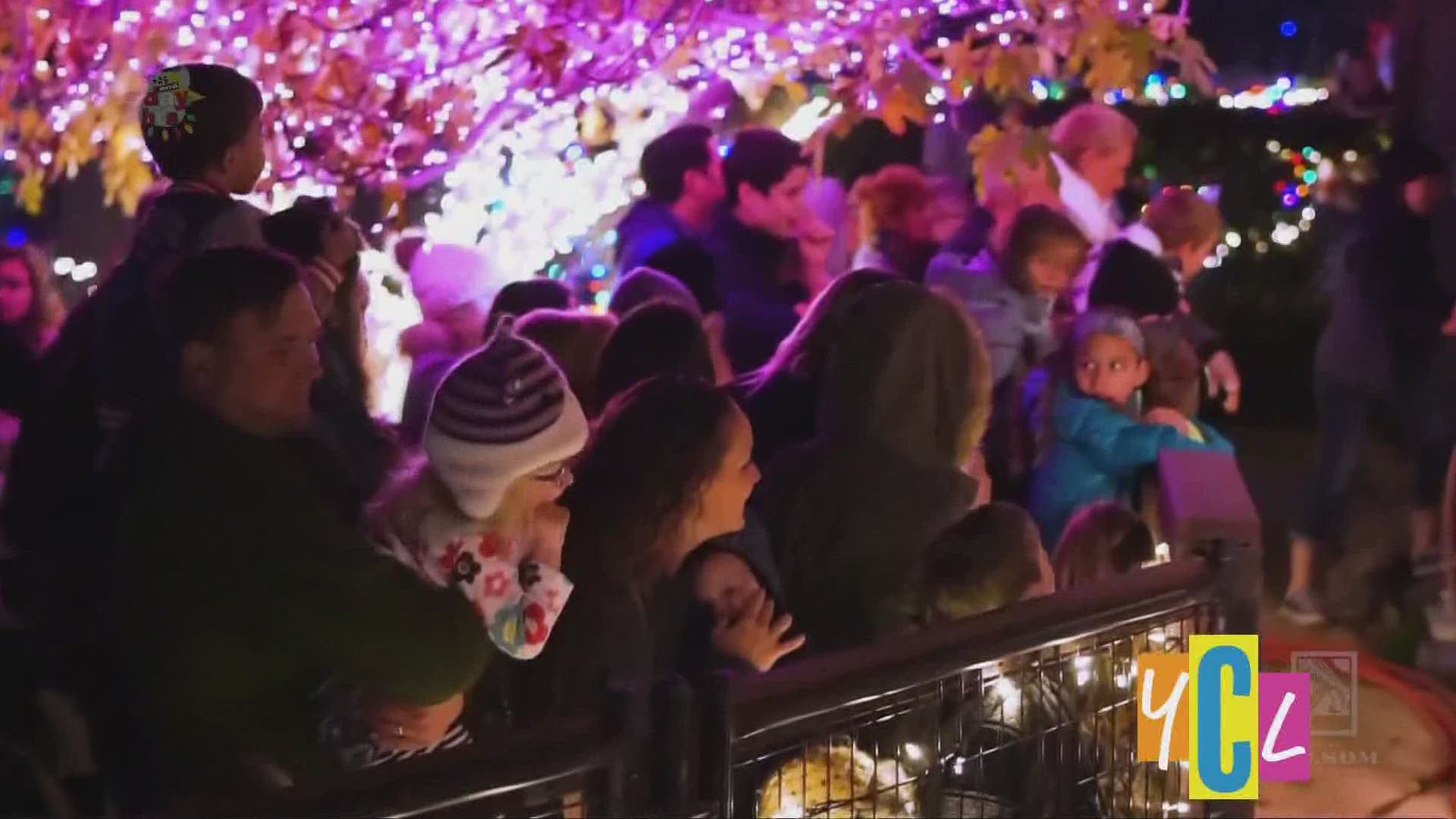This nighttime photograph captures a bustling crowd gathered outdoors, likely celebrating a holiday festival of lights. The image is taken from a slightly elevated angle, looking down at the diverse group of people. They are bundled up in winter clothing, with many wearing jackets and beanies to fend off the cold. The crowd, which includes various genders, ethnicities, and age groups—from babies and toddlers to older children—stands behind a brown metal fence with an open fretwork design. Some parents have their children on their shoulders to provide a better view. Everyone in the crowd appears to be looking toward the upper right corner of the photo.

In the background, a large tree adorned with small white Christmas lights casts a subtle, enchanting glow that lends a pink hue to the scene. Various light sources further illuminate the area, contributing to the festive atmosphere. In the bottom right corner of the image, the letters "YCL" are prominently displayed in an artistic manner: the "Y" is in white on an orange background, the "C" is in blue on a yellow background, and the "L" is in white on a pink background.